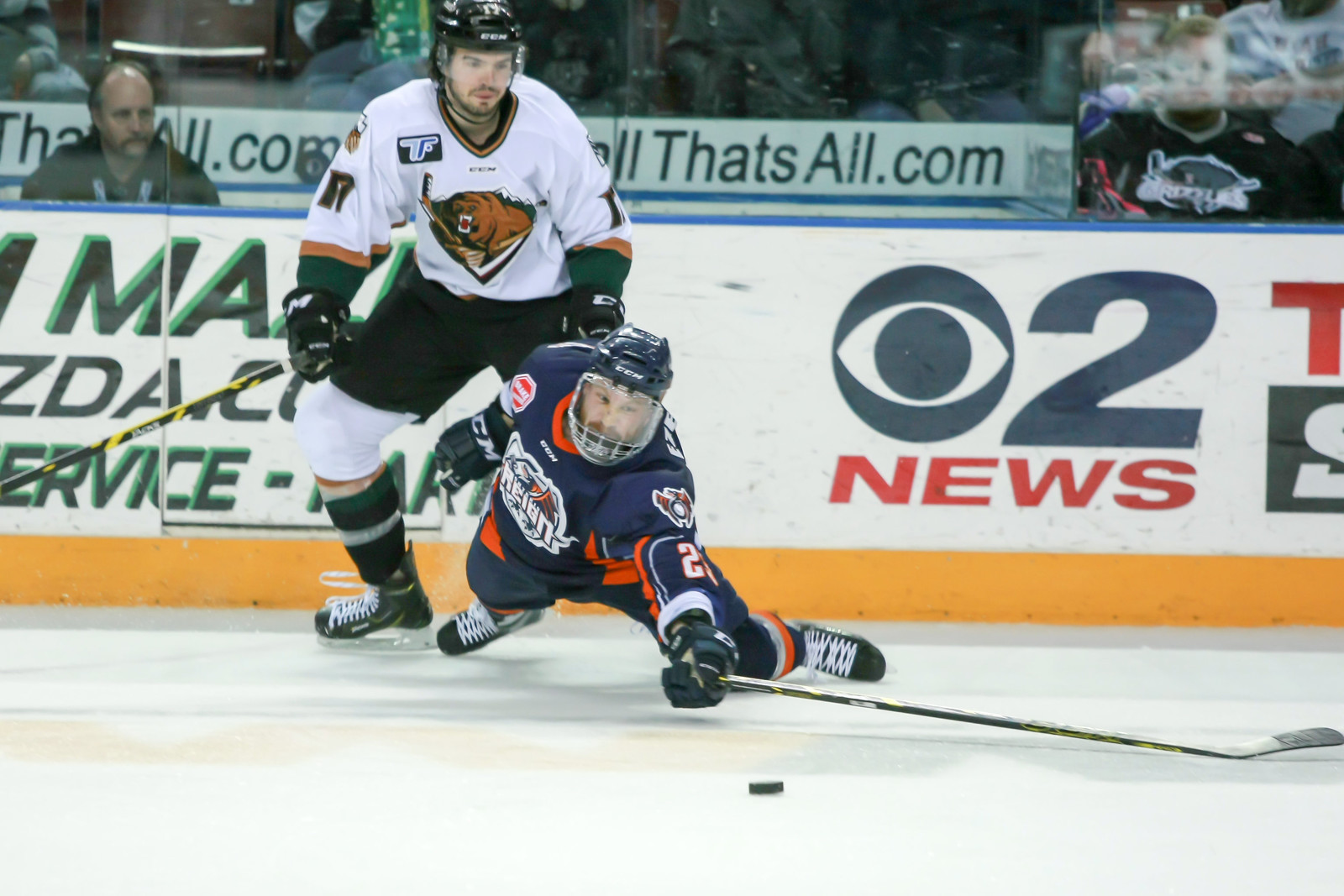This action-packed photograph captures an intense moment in an ice hockey game, focusing on two players on the ice. Dominating the scene in the foreground, one player in a dark blue uniform with white and orange trim and a matching helmet appears to be lunging or nearly falling, desperately reaching out with his black hockey stick for the puck. The puck itself is located towards the bottom center-right of the frame. Just behind him stands another player donned in a white jersey with black and brown trim, black shorts, and white and black gear below the shorts. This player seems to be strategizing his next move as he fixes his gaze on the puck. In the background, the white rink walls feature various colorful sponsorship graphics and an orange band runs along the bottom where the ice meets the wall. Beyond the rink walls, spectators can be seen seated behind a plexiglass barrier, intently watching the high-stakes action unfold on the ice.